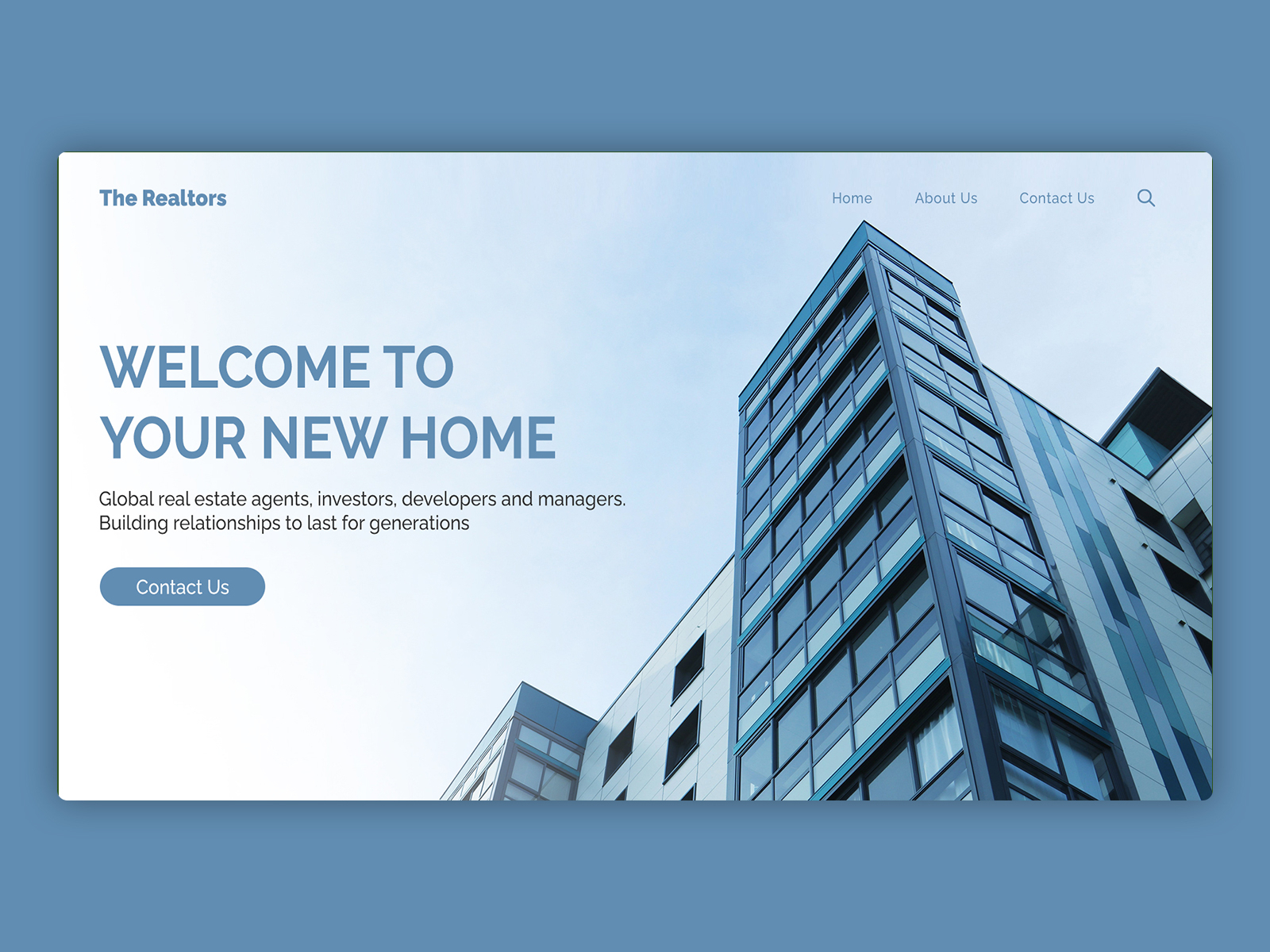The image consists of a horizontally oriented blue rectangle that forms the background. The shade of blue is a dusty medium tone. Embedded on top of this is a slightly smaller rectangle containing a photograph of a building, with the photograph almost reaching the edges on the right and left sides, but with noticeable margins at the top and bottom. The perspective of the photograph is from a close-up, upward angle, and shows the building dominating the right side of the image while the left side features mostly sky. The building appears to have multiple windows on its facade and the entire photograph is tinted in blue shades, giving a monochromatic look.

Overlaying the photograph, the top-left corner displays the word "Realtors" in white text. Aligned horizontally on the same level, towards the right side, are links labeled "Home," "About Us," "Contact Us," and a magnifying glass icon, presumably for search functionality.

Prominently placed in the center-left of the photograph is the main headline, "Welcome to your new home," written in a bold, dark blue font that matches the background color. Directly beneath this, in smaller black text, is a tagline reading "Global real estate agents, investors, developers, and managers build relationships to last for generations." Below this tagline is a blue "Contact" button that blends seamlessly with the background color. The overall color palette of the image, including the fonts and button, predominantly features different shades of blue, with the text and clouds providing contrast for legibility and emphasis.